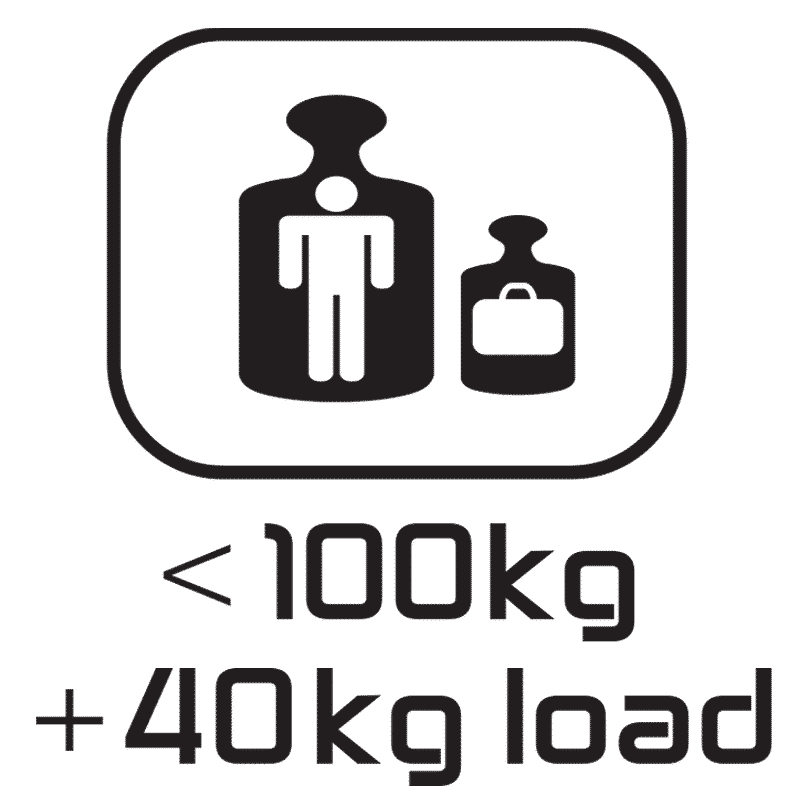The image is a black and white informational graphic set against a white background, possibly intended as a sign for an airport. It features two black outlined shapes resembling perfume bottles. Within the larger bottle on the left is a minimalist, white silhouette of a man, characterized by a circular head and squarish body, akin to the generic restroom symbol for men. To the right, in a smaller bottle, is a white silhouette of a suitcase or briefcase. Below these shapes, large text provides details: a less than symbol next to "100 kg" on the top line, and a plus sign followed by "40 kg load" on the bottom line, indicating permissible weight limits. The overall design is simple, with solid graphics and text, devoid of shading or complex details.